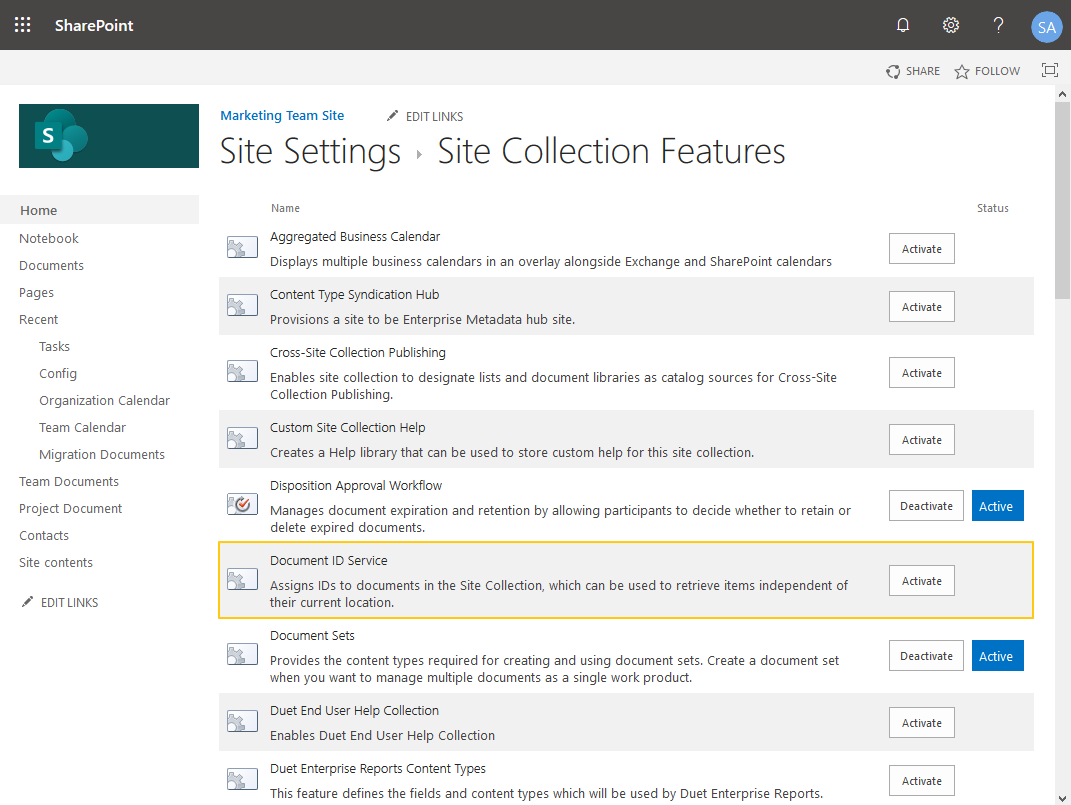The image portrays a SharePoint interface page with a comprehensive layout and various navigational elements. At the top, a gray or black bar features the SharePoint logo in the upper left corner, while the upper right corner hosts a series of buttons including notifications, settings, a help question mark, and a user icon displaying the initials "SA." 

Beneath the top bar, the interface is sectioned into various navigation elements. On the left side, there is a vertical menu with several options including Home (currently selected), Notebook, Documents, Pages, Recent, Tasks, Config, Organization Calendar, Team Calendar, Migration Documents, Team Documents, Project Document Contacts, and Site Contents. At the bottom of this menu, there's an Edit Links option.

On the main part of the page, to the right, prominent headings such as "Marketing Team Site," "Edit Links," "Site Settings," and "Site Collection Features" are visible. Below these headings, the page details various features that can be activated. 

Specifically, the "List" section mentions an Aggregated Business Calendar, which can display multiple business calendars alongside Exchange and SharePoint calendars. The Document ID Service within this list is notably highlighted with a yellow border, emphasizing its importance or indicating that it is currently selected. Additional features listed include Content Type Syndication Hub, Cross-Site Collection Publishing, Custom Site Collection Help, Disposition Approval Workflow, and Document Sets, among others, each accompanied by an "Activate" button.

Notably, two of the items, Document Sets and Disposition Approval Workflow, are currently deactivated and need activation, highlighting their immediate requirement for user action.